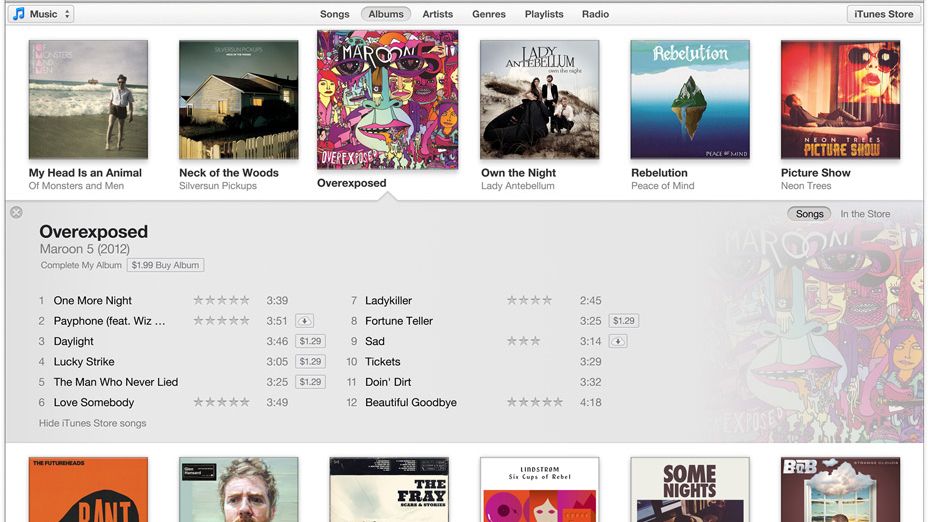The image depicts an older version of iTunes on a computer screen, showcasing a variety of music options. The primary background of the interface is a clean white and gray. In the top left corner, there is a small blue music symbol, followed by the word "Music" in black text. Confirming this is indeed iTunes, the top right corner displays "iTunes Store."

In the top center of the screen, various categories are visible, including Songs, Albums, Artists, Genres, Playlists, and Radio. The "Albums" category is currently selected. Several albums are prominently displayed at the top of the screen, each featuring its album cover with corresponding black text beneath.

From left to right, the albums showcased are:
- "My Head is an Animal" by Of Monsters and Men
- "Neck of the Woods" by Silversun Pickups
- "Overexposed" by Maroon 5
- "Own the Night" by Lady Antebellum
- "Rebellion" by Peace of Mind
- "Picture Show" by Neon Trees